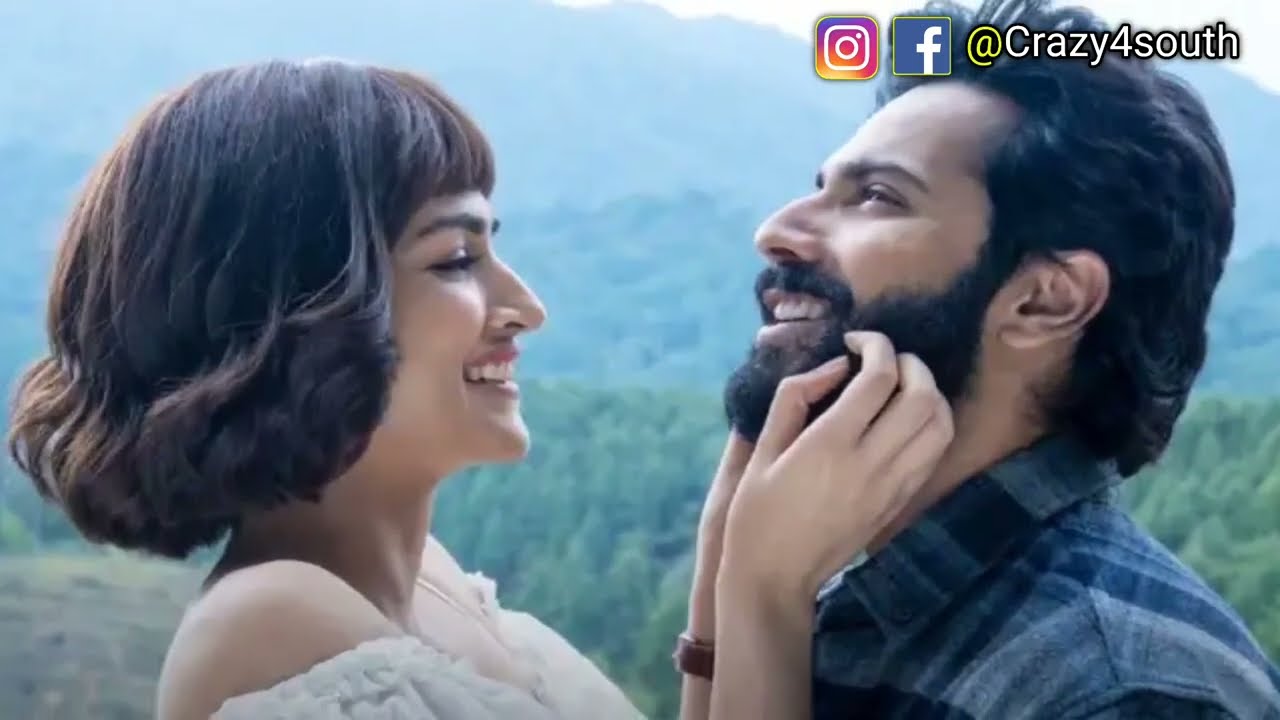In this close-up shot, a medium-skinned woman with shoulder-length, slightly curly brown hair styled in a bob, is playfully running her fingers through a medium-skinned man's wavy black hair and dense black beard. She is smiling brightly, wearing a white strapless dress, a pearl necklace, and a watch with a brown leather strap on her left wrist. The man, wearing a dark gray and blue plaid shirt, has his head slightly tilted back, looking up above her with a grin on his face. Above their heads, the Instagram and Facebook logos are visible alongside the handle @crazy4south. They are positioned in front of a blurry background of forested mountains, adding a scenic touch to the affectionate moment.